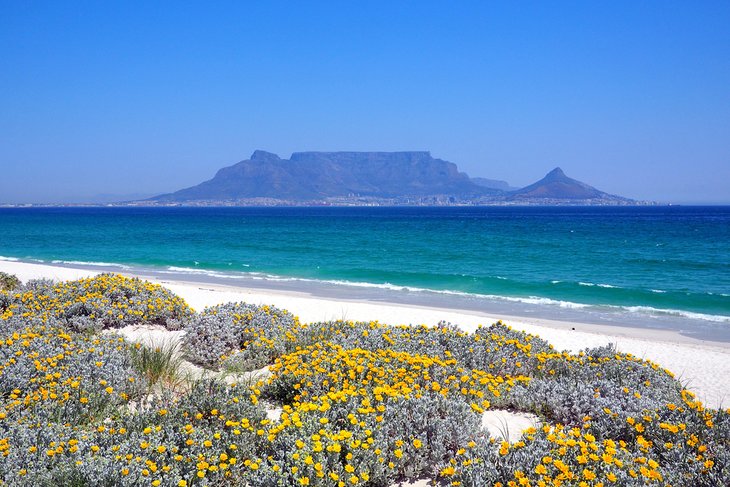This captivating photograph depicts a serene beach scene under a bright blue sky, characteristic of a sunny day. The sandy shore, a light shade of beige, is dotted with clusters of vibrant orange and yellow flowers, growing amidst grayish bushes and sparse vegetation. Glancing beyond the beach, the teal-colored ocean displays a striking gradient, transitioning from a light, bright teal in the foreground to a deeper, darker blue further out. Dominating the horizon, a prominent landmass rises from the sea, resembling a large island with distinct rock formations that evoke the shape of cliffs or volcanic cones. The island's shoreline features architectural structures that add a touch of human presence to this naturally picturesque landscape.